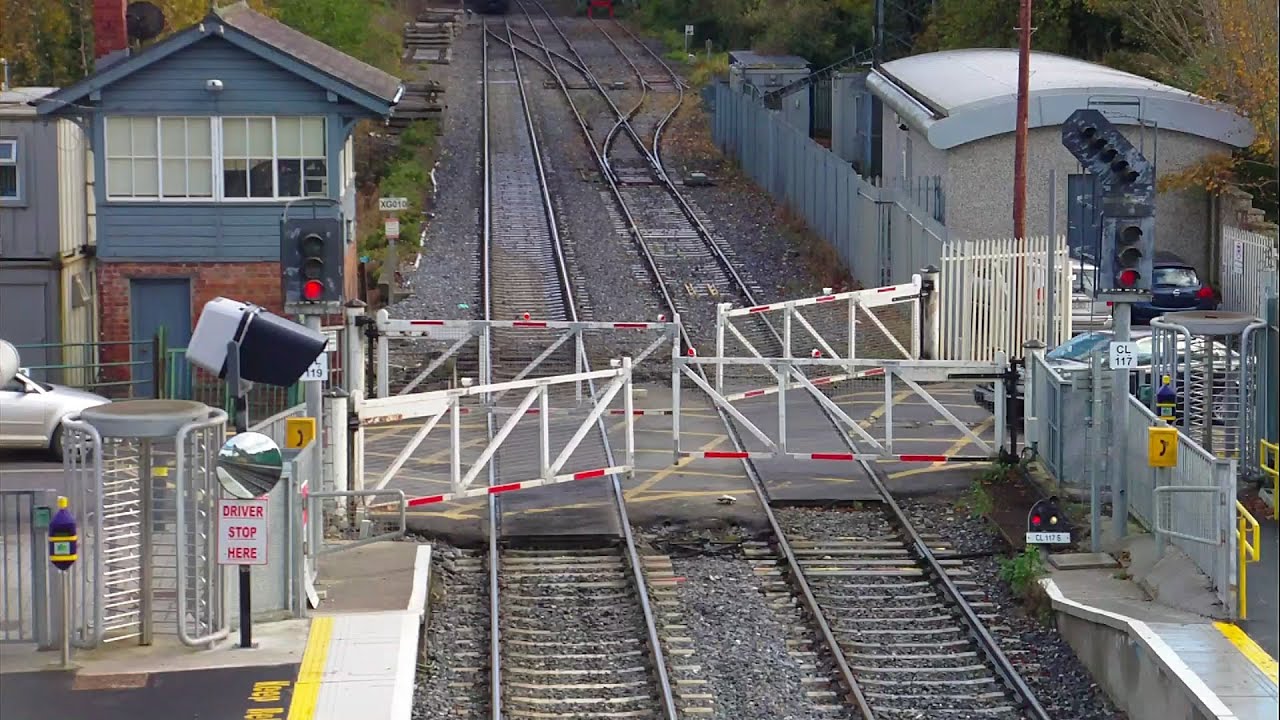This horizontally aligned rectangular picture, taken at a slight downward angle, captures a daytime scene of a railroad crossing with two sets of train tracks running through the center. The tracks extend towards the top of the image, veering off in different directions. On the left side, there is a two-story building that resembles a house, featuring a brick lower level, a blue door, blue-painted sidings, and a black hipped roof. Behind it stands another older, beige two-story building. To the right, there is a short stone building with a curved white roof. A train signal and stoplight are mounted on a pole on the right side of the tracks. The railroad crossing is framed by black or dark gray sidewalk with yellow stripes. Both sides of the tracks have white railroad fencing, and the gates, presently open, allow cars to pass through. A black car is seen entering from the right side of the frame. The red lights of the railroad signals indicate that passage is currently blocked for trains, and a "driver stop here" sign is visible to the left. There are also cars parked along the streets on either side of the tracks, which suggests intersections with additional roads leading to the train station.